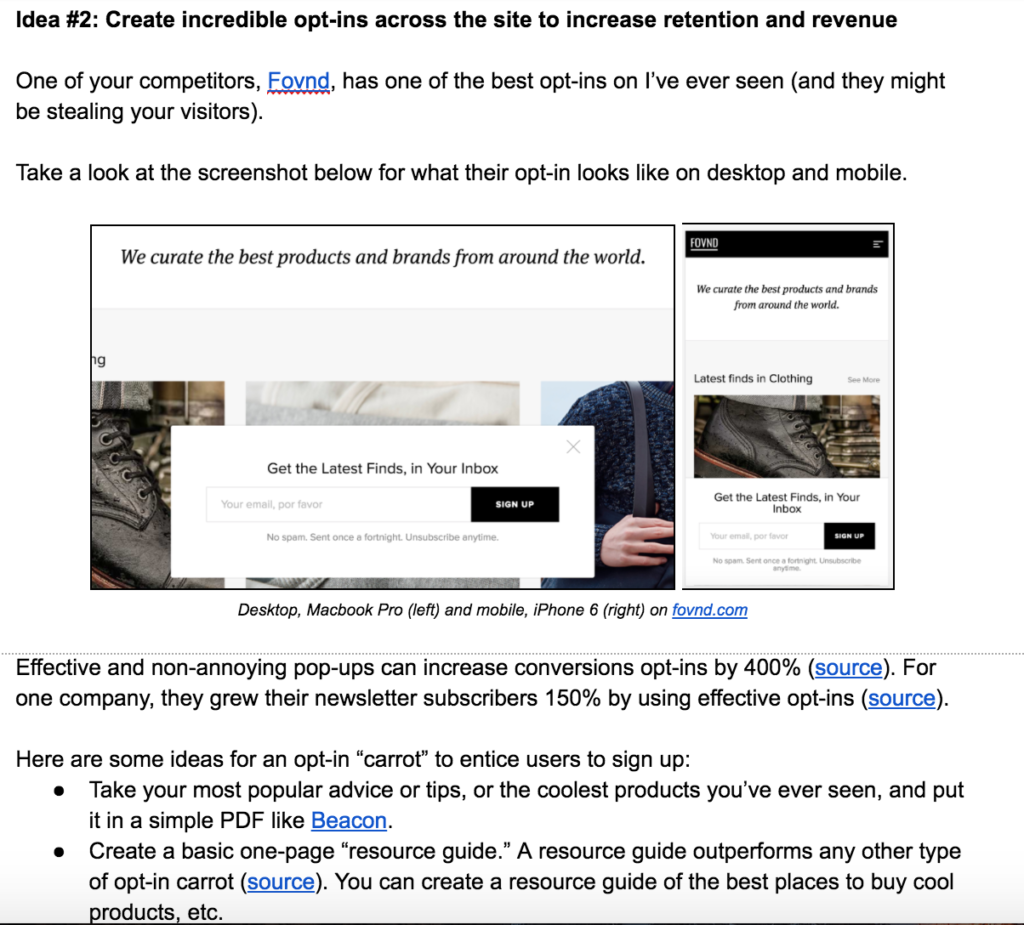The image features a substantial amount of black text against a white background, interspersed with screenshots from both a desktop and a mobile device. At the top, in bold black text, the heading reads: **"Idea Number Two: Create Incredible Opt-Ins Across the Site to Increase Retention and Revenue."**

Beneath this heading, in regular black text, it states: "One of your competitors, **F-O-V-N-D**" (with the name written in blue), "has one of the best opt-ins I’ve ever seen and they might be stealing your visitors" (with the latter part in parentheses). 

The following sentence instructs readers to examine the provided screenshots for examples of what their competitor's opt-in looks like on both desktop and mobile devices.

The first screenshot, in landscape orientation, showcases a desktop view. It features the text: "We curate the best products and brands from around the world," displayed in black on a white background. Below this is a pop-up asking users to "Get the latest finds in your inbox," accompanied by a text field for an email address and a black sign-up button.

Next to it, the second screenshot mirrors the content, but from a mobile view. It also displays the text: "We curate the best products and brands from around the world," and features an identical pop-up window prompting users to enter their email address to receive updates.